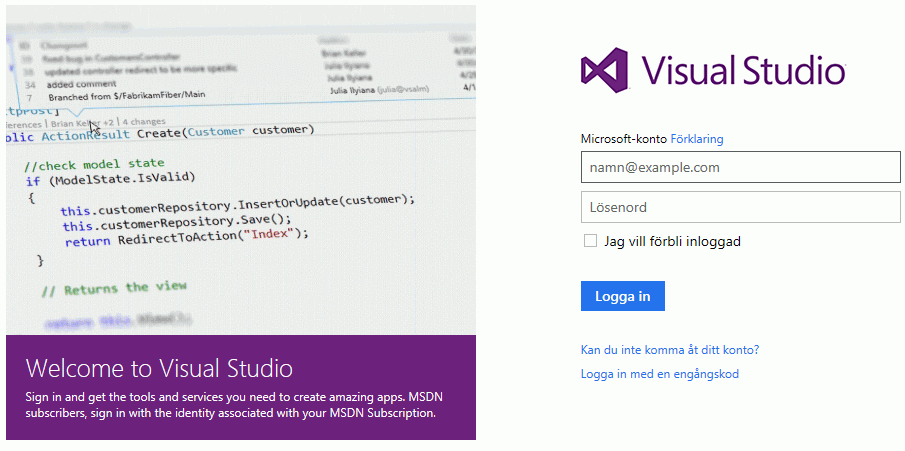The horizontally rectangular image is divided into two sections. On the left side, at a diagonal angle, there is a screenshot of a coding website, featuring some written code. Beneath this, a horizontally rectangular purple banner displays the message: "Welcome to Visual Studio. Sign in and get the tools and services you need to create amazing apps. MSDN subscribers, sign in with the identity associated with your MSDN subscription."

On the right side, against a white background, the Visual Studio logo is prominently placed at the top. Below the logo, there is a sign-in area in a foreign language. Despite this, the layout suggests that the top field is for the email address and the field below is for the password. A blue login button below these fields is labeled "LOGGA in." Additionally, there are two lines of text underneath the button that appear to be hyperlinks, although they are written in a language other than English.